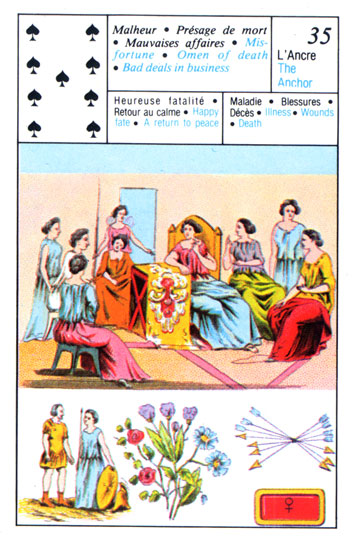In the image, the focal point is a playing card placed in the upper left corner, set against a white background. This card features a series of black spades—four on one side, one in the center, and another four on the opposite side. Adjacent to this card, there is a black box containing text written in blue that reads: "Misfortune, omen of death, bad deals on business." Below this box, two smaller squares contain additional blue text: "Happy fate, a return to peace," and "Illness, wounds, and death."

In the upper right corner of the image, there is a small square with the number 35 and the word "The Anchor" written in blue text. Beneath it, in black text, is the word "L'ANCRE."

Dominating the central area of the image is an illustration of a group of women. They are all seated and dressed in long dresses with short, dark hair. One prominent woman sits in a chair with a very tall gold back, resting her arm on a table covered with a gold and red tablecloth. Another woman in the background, wearing a pink shirt, appears to have wings on her back.

In the bottom section of the image, a man and woman dressed in medieval attire stand beside each other. Around them, there are various elements—a bouquet of flowers, crossing arrows, and a red rectangle featuring a female symbol.